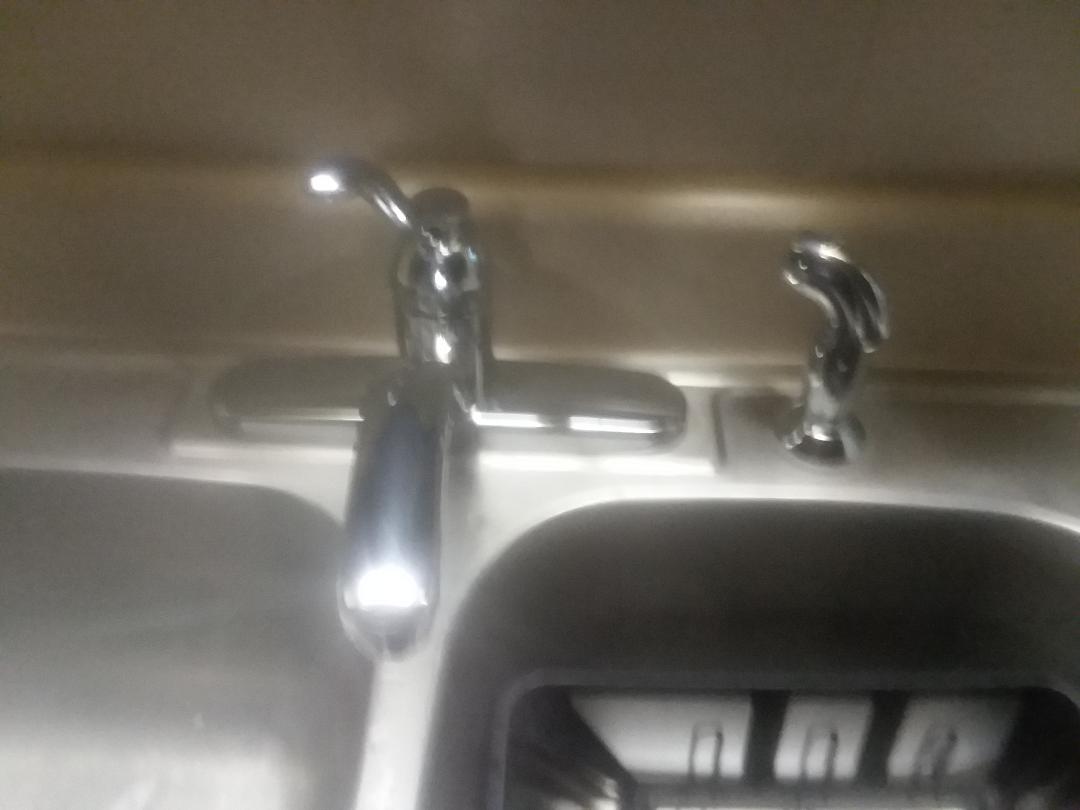This blurred photograph showcases a shiny, stainless-steel kitchen sink with a dual-compartment design. The main feature is the silver faucet with a single swiveling handle that allows adjustment of water temperature by turning left or right. Adjacent to the faucet, there is a matching silver pull-out spray nozzle positioned on the right side. The sink, brightly illuminated by a strong light source, possibly daylight, casts glaring reflections due to its polished surface.

The sink comprises two sections: the left compartment appears empty, intended for washing, while the right compartment contains a black plastic dish strainer. The background is a beige or tan-colored wall, contributing to a neutral ambience. Above the sink, there's an unclear presence of a tile or solid backsplash area, adding to the kitchen setting. Despite the image’s grainy and out-of-focus nature, the predominant colors are silver, black, beige, and tan, forming a modern look with a mix of shiny and brushed textures.